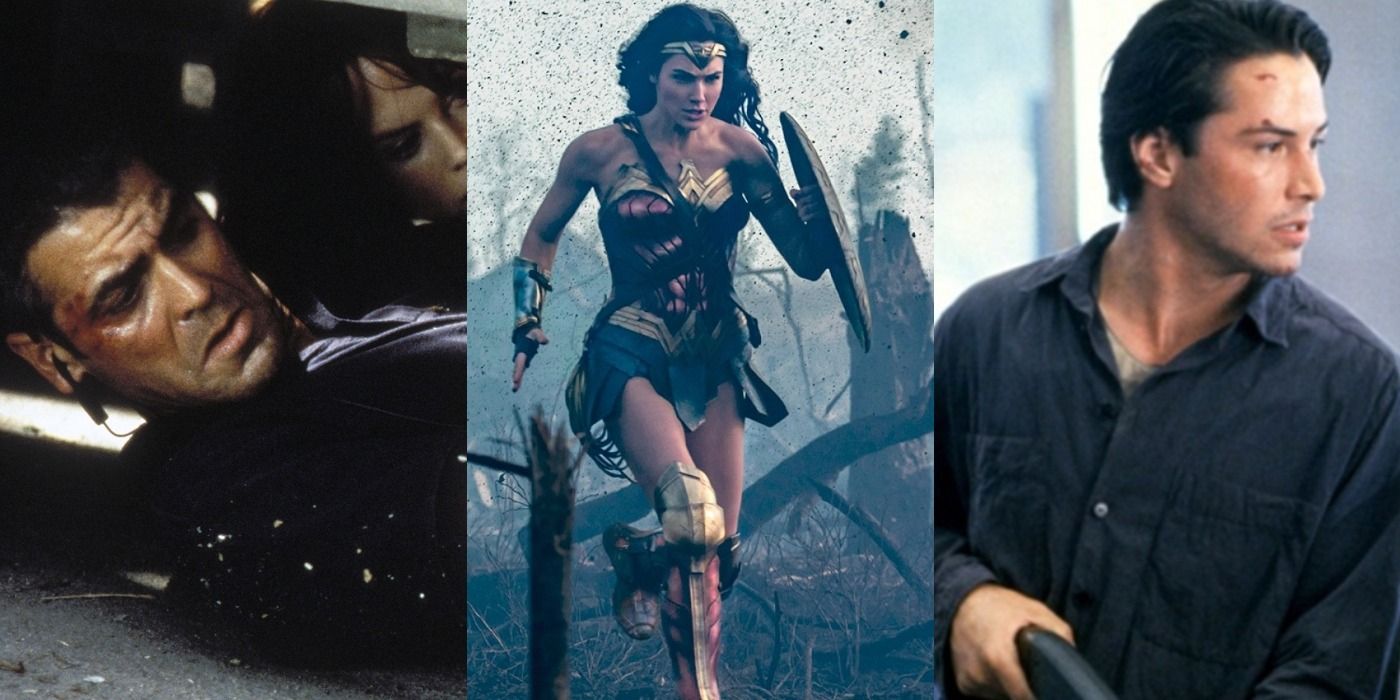This composite image features three distinct scenes placed side by side in a collage. On the left, we see a tense moment where George Clooney and a woman, possibly his co-star, are lying down under some form of shelter. Clooney, captured from the bust up, has a bruise on the side of his head, slightly above his right eye, and wears an earpiece. Both characters seem focused on something to the right, amidst a background strewn with rubble.

The center image showcases Gal Gadot as Wonder Woman, running vigorously with her shield held aloft in her left hand. She is clad in her iconic costume: predominantly red armor with golden and blue accents, which includes her chest armor, gauntlets, and boots, although parts of her arms, thighs, and head remain exposed. With her long black hair flowing behind her, she charges through a chaotic landscape littered with debris, fallen trees, and destroyed buildings, suggesting the aftermath of a battle.

On the right, Keanu Reeves, possibly in a scene from the John Wick series, directs his gaze to the left. His short, slicked-back black hair frames a face marked by a cut above his right eyebrow and another along his forehead. Dressed in a long-sleeved black button-up shirt over a gray undershirt, Reeves holds what appears to be a rifle in his right hand, contributing to the action-oriented vibe of the trio of images.